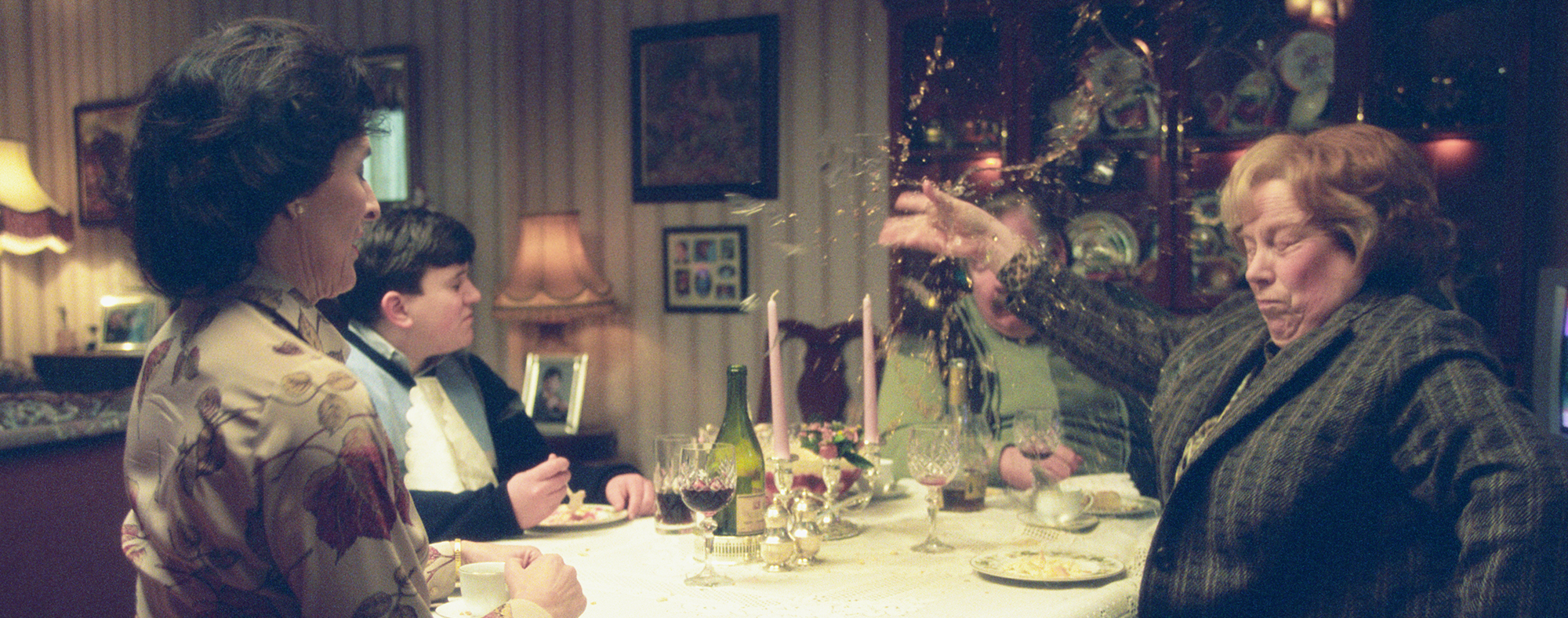In this image, a family is gathered around a dinner table set with plates, wine glasses, and pink candles. The background is adorned with striped patterns. Seated at the table, we have a woman on the right who appears to be wearing a suit jacket; she seems to be dancing while in her seat. Beside her, a man and a boy with straight black hair are also present. The boy is focused on his plate. On the far left, yet another woman is included in the scene. The image captures a dramatic moment where the woman in the suit jacket has thrown or broken a glass, causing shards to fly and resulting in a mix of confused and angry reactions from those around her. The lighting in the room enhances the vividness of the scene, emphasizing the surprised expressions and the chaotic atmosphere at the table.